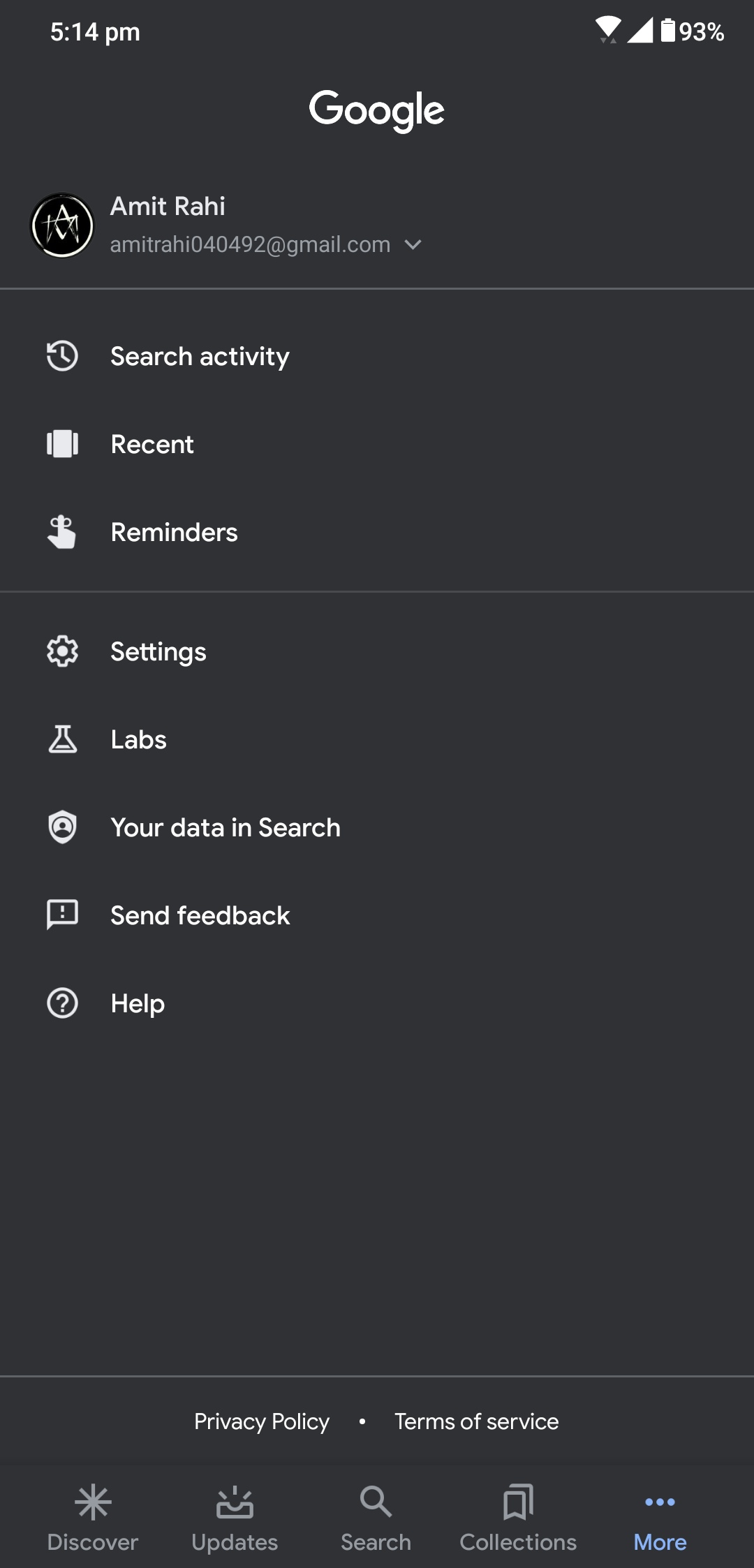In this image, someone is browsing their Google account settings on a smartphone. The screen displays a clear and medium-toned background. At the top left corner of the screen, the time reads 5:14 PM in white font. On the right side of the top bar, various status indicators are visible, showing battery life at 93%, signal strength, and other connectivity icons.

Centered at the top is the bold, white Google logo. Below the logo, the user’s profile information is displayed. The profile picture shows the initials "A M" for Amit Rahi, and the email address "amitrahi040492@gmail.com" is listed in thin, light gray text.

Under the profile section is the heading "Recent Reminders," with small icons to the left for easy identification. Further down, a light gray line separates this section from the subsequent options, which are listed as "Settings," "Labs," "Your data in Search," "Send feedback," and "Help," each accompanied by their respective Google icons.

At the bottom of the screen, another light gray line appears, followed by the terms "Privacy" and "Terms of Service." Finally, at the very bottom, a menu bar features various navigation options: "Discover," "Updates," "Search," "Collections," and "More." The "More" option is highlighted in light blue, while the other options are displayed in light gray. Each option is paired with a relevant icon, such as a star, an inbox, a magnifying glass, and bookmark symbols.